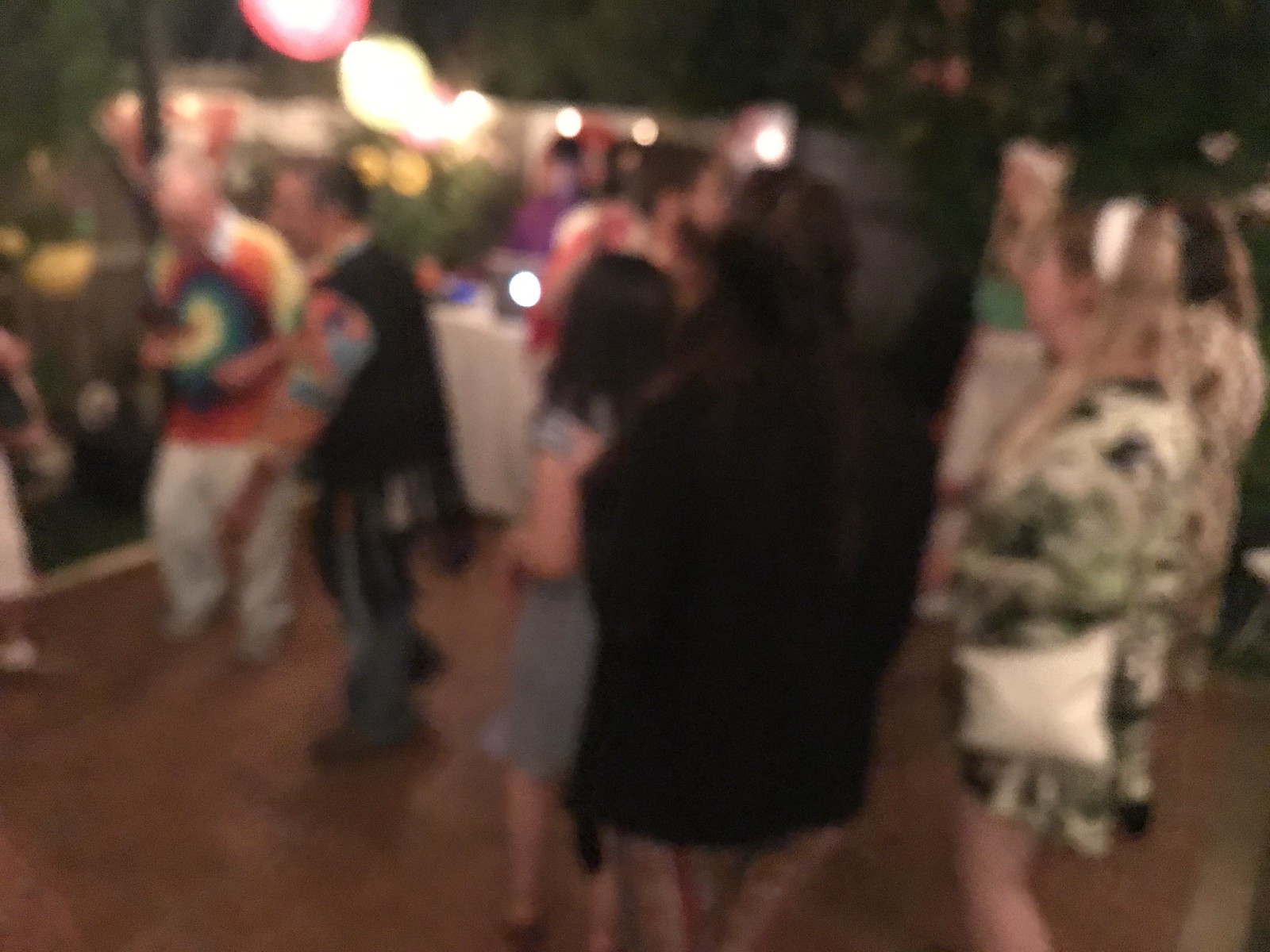The photograph depicts a lively nighttime outdoor party, albeit captured in a blurry manner that obscures finer details. The horizontal, rectangular image features a mix of colorfully dressed attendees, suggesting a celebratory atmosphere. Central to the scene is a white table adorned with snacks and refreshments, emphasizing the social nature of the gathering. The background reveals a dark sky, possibly indicating an outdoor setting under a pergola-like structure, with an assortment of hanging lights, including a prominent red light in the center transitioning to white lights near what may be a house. To the back left, green bushes and a white wall add to the environment's ambiance.

In the foreground, a light brown floor, likely a dance floor, hosts several dancing individuals. A man on the left in a vibrant tie-dye shirt featuring hues of yellow, green, blue, red, and orange pairs his outfit with white pants, seemingly captured mid-dance. Beside him, another man dons a colorful shirt layered with a black vest. On the right side of the image, a woman in a green and white dress with a white shirt and headband stands out, along with a group of four women whose backs are turned to the camera, enhancing the social gathering's dynamic. Despite the image's blurriness, the festive decorations, including yellow and pink balloons and sparkling lights, along with the diverse attire of attendees, depict a joyful and energetic celebration.